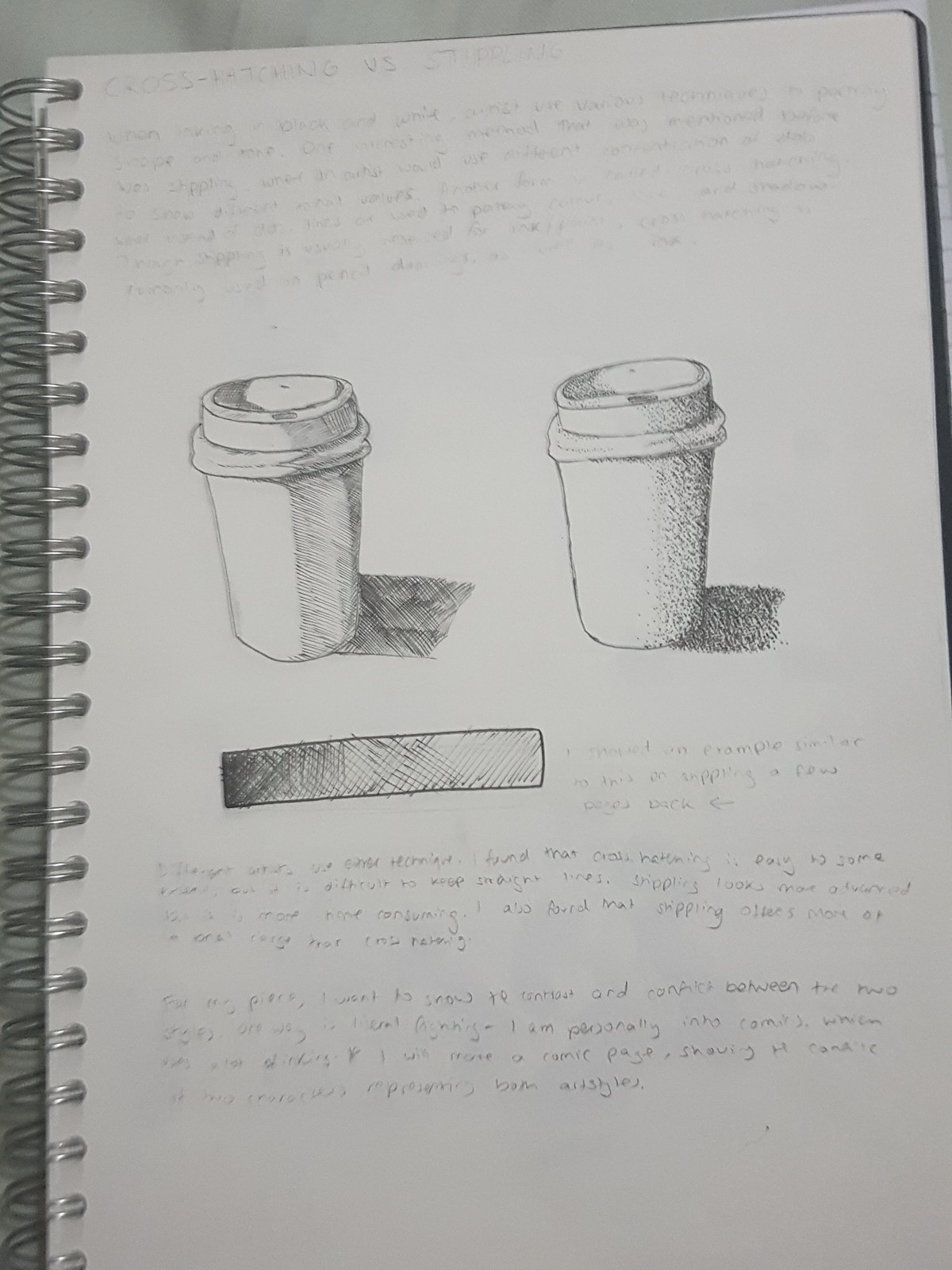The image features a page from a spiral-bound art book containing a detailed pencil sketch. The sketch depicts two reusable coffee cups, placed side by side. The cup on the right is designed with hexagonal facets, whereas the cup on the left has a smooth, cylindrical shape. The right-hand cup casts a longer, more pronounced shadow, while the left-hand cup's shadow is shorter and less defined. Scattered around the sketch are faint, handwritten notes in pencil, though the text is largely difficult to discern due to its faded nature. One legible snippet reads, "creativity is easy to some." Another partially visible phrase suggests something about shipping but remains mostly undecipherable. Despite the faded text, the intricate details of the pencil work and shadow contrast between the two cups stand out vividly.